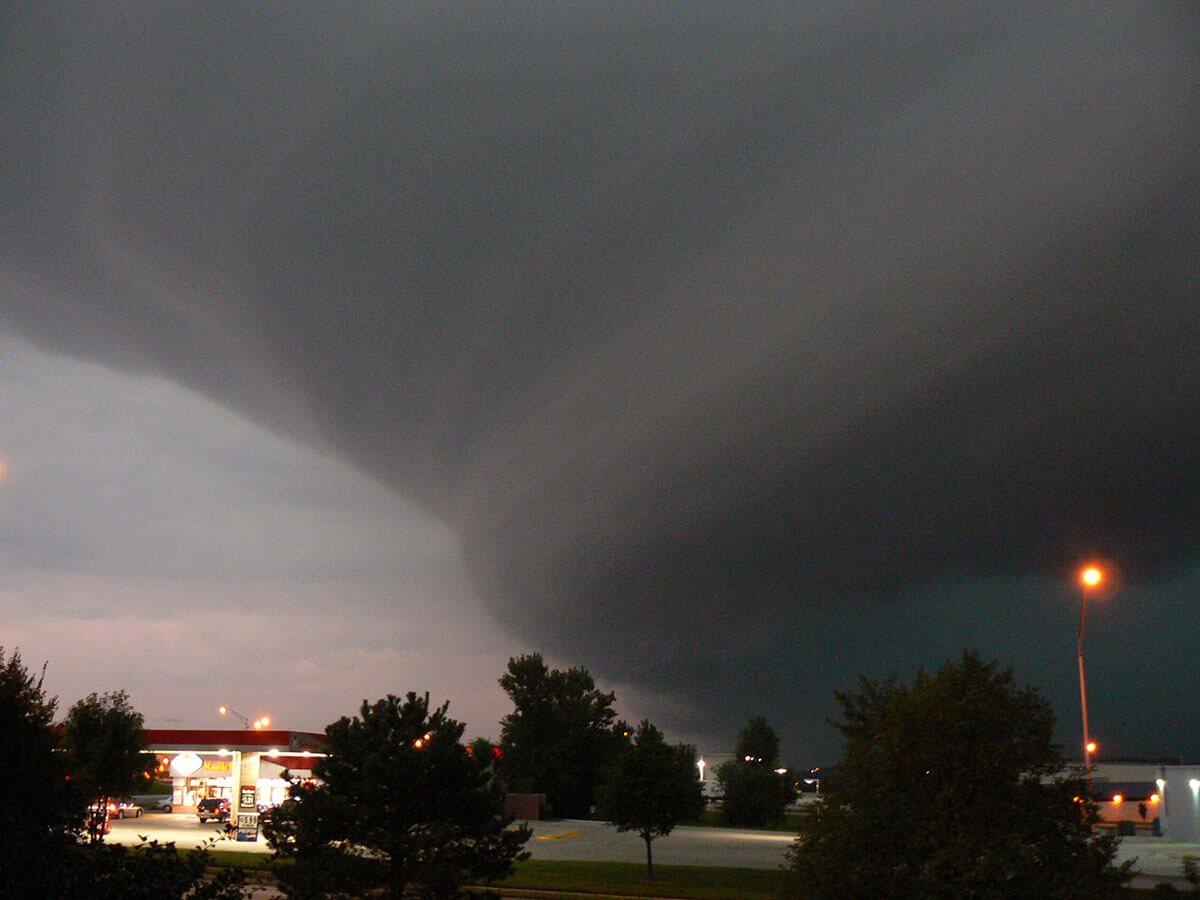This photograph captures a dramatic tornado-like storm cloud looming ominously over a cityscape. The entire sky is dominated by a massive, dark gray cloud formation spiraling downward, creating an intense funnel shape that descends towards the ground. The scene is set at dusk, with the upper part of the sky entirely consumed by the swirling storm, while the lower edge reveals a sliver of transitioning daylight with hints of blue and pink hues. Below the menacing cloud, a small city area is visible, featuring a well-lit gas station with a red roof and white walls on the left side of the picture. Adjacent to the gas station is a roadway flanked by trees. Various buildings with illuminated windows are situated directly under the menacing formation. An orange street light glows on the bottom right corner of the image, adding to the eerie ambiance. The overall lighting suggests a somber twilight, highlighting the stark contrast between the approaching storm and the city's tranquil illumination.